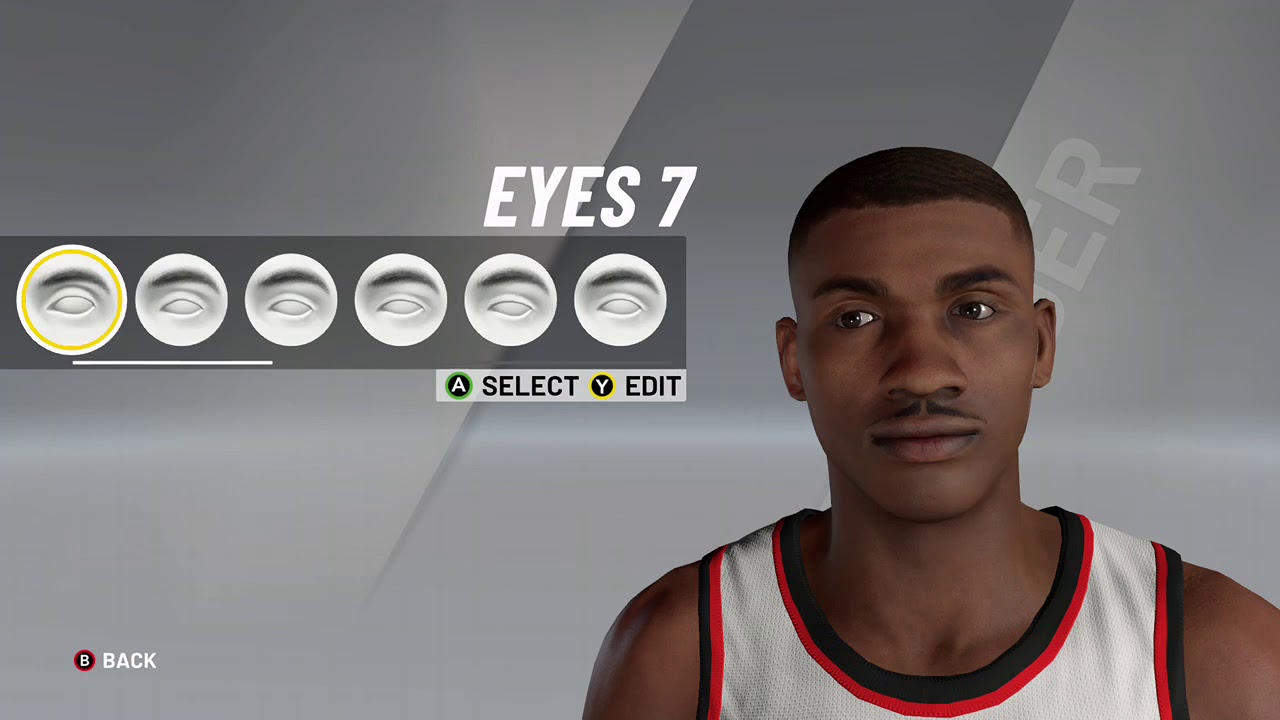In this image, we see a detailed customization page for a character in an NBA video game. The character customization interface allows users to tailor various aspects to suit their preferences. The prominent colors in the interface are black, white, and red, giving it a sleek, sports-themed feel. On the bottom left of the screen, there's a back icon for returning to the previous menu. Additionally, select and edit buttons are available for making specific changes. The current focus of the menu is on editing the eyes of the character, offering options to adjust their appearance precisely.